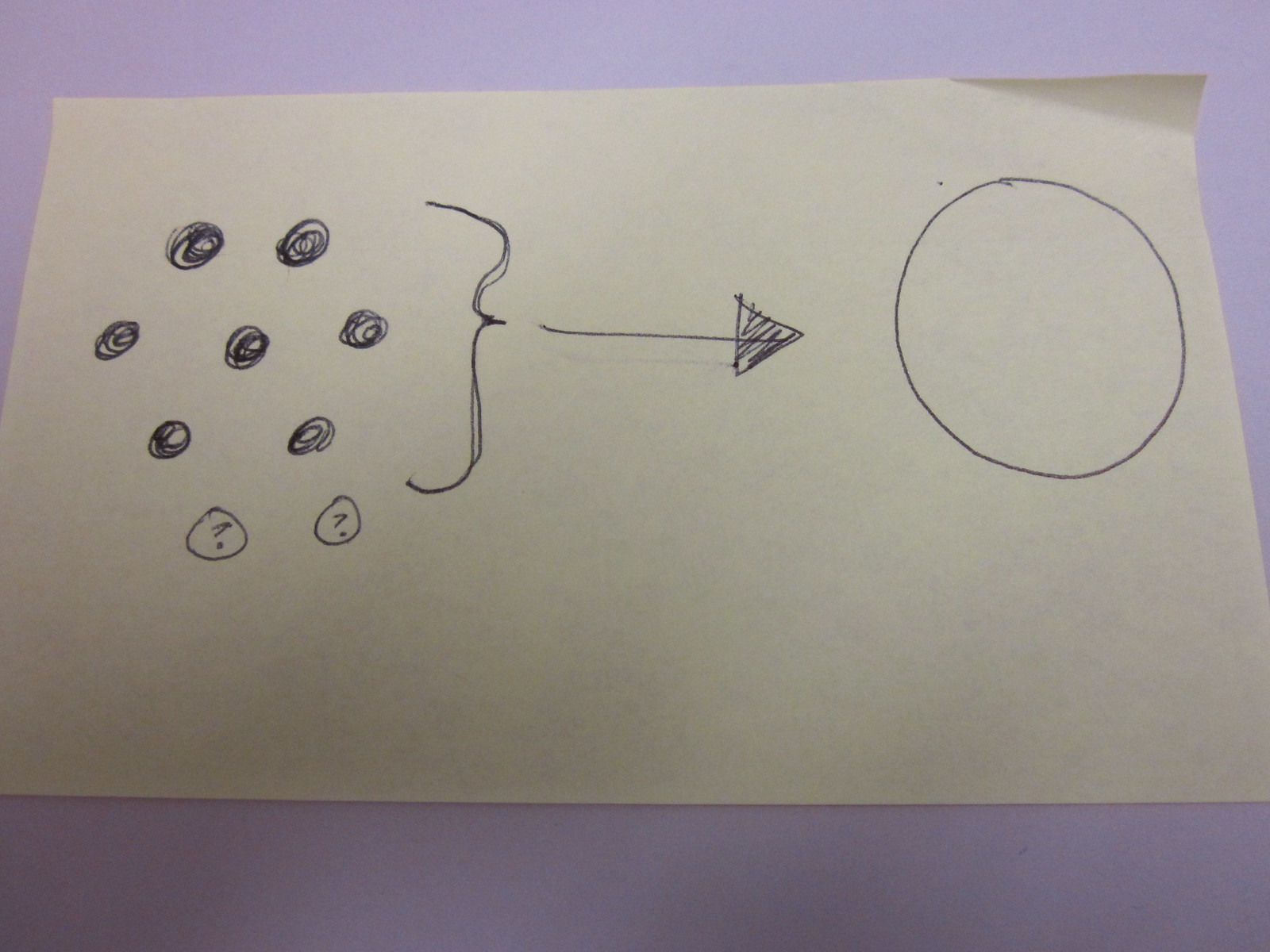This image features a hand-drawn diagram on a piece of paper with a soft lavender background. The paper itself is an off-white, grayish tone resembling doodle paper, and the top right corner is slightly bent. The diagram is rendered in black ink, not ballpoint pen. 

On the left-hand side of the paper, there are seven fully colored-in circles stacked vertically. Below these circles, there are two additional circles, each containing a question mark. To the right of this arrangement, a parenthesis symbol leads into an arrow that is partially filled in with scribbles, directing attention to the right. The arrow points towards a nearly perfect, empty circle drawn with meticulous precision. 

The diagram appears to illustrate a transformation or equivalence, suggesting that the seven filled circles and the two questioned circles collectively evolve into or equal this singular, flawless circle. The overall composition is intriguing and thought-provoking, complemented by the visually pleasing lavender background that enhances the presentation.